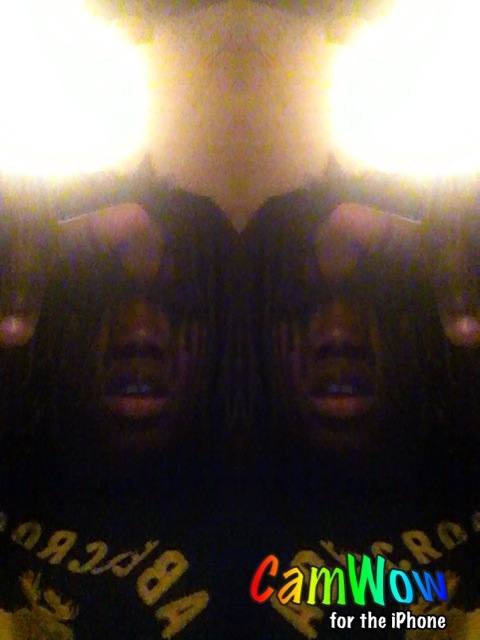The image depicts a low-quality, grainy, digitally manipulated photograph that appears to have been taken with a low-quality iPhone camera. The watermark in the bottom right corner, which reads "CAM WOW" in rainbow-colored letters progressing from red to blue, indicates that special effects were used. Below this, the text "FOR THE IPHONE" is written in white with a black outline. The image primarily features a young black male with black dreadlocks that fall over his face. He is wearing what appears to be a dark navy blue shirt with yellow or gold print, possibly from Abercrombie. The photograph is a duplicated mirror image of the boy, creating a side-by-side effect with his mouth open and teeth showing. He seems to be looking at the camera, with his thumbs visible in an up gesture, though one person mentioned it might be his middle finger, it's unclear because of the poor quality. The entire image is heavily overexposed at the top, giving the appearance of two orbs of whitish-yellow light flanking a vaguely visible neck, enhancing the eerie and surreal quality of the photograph.